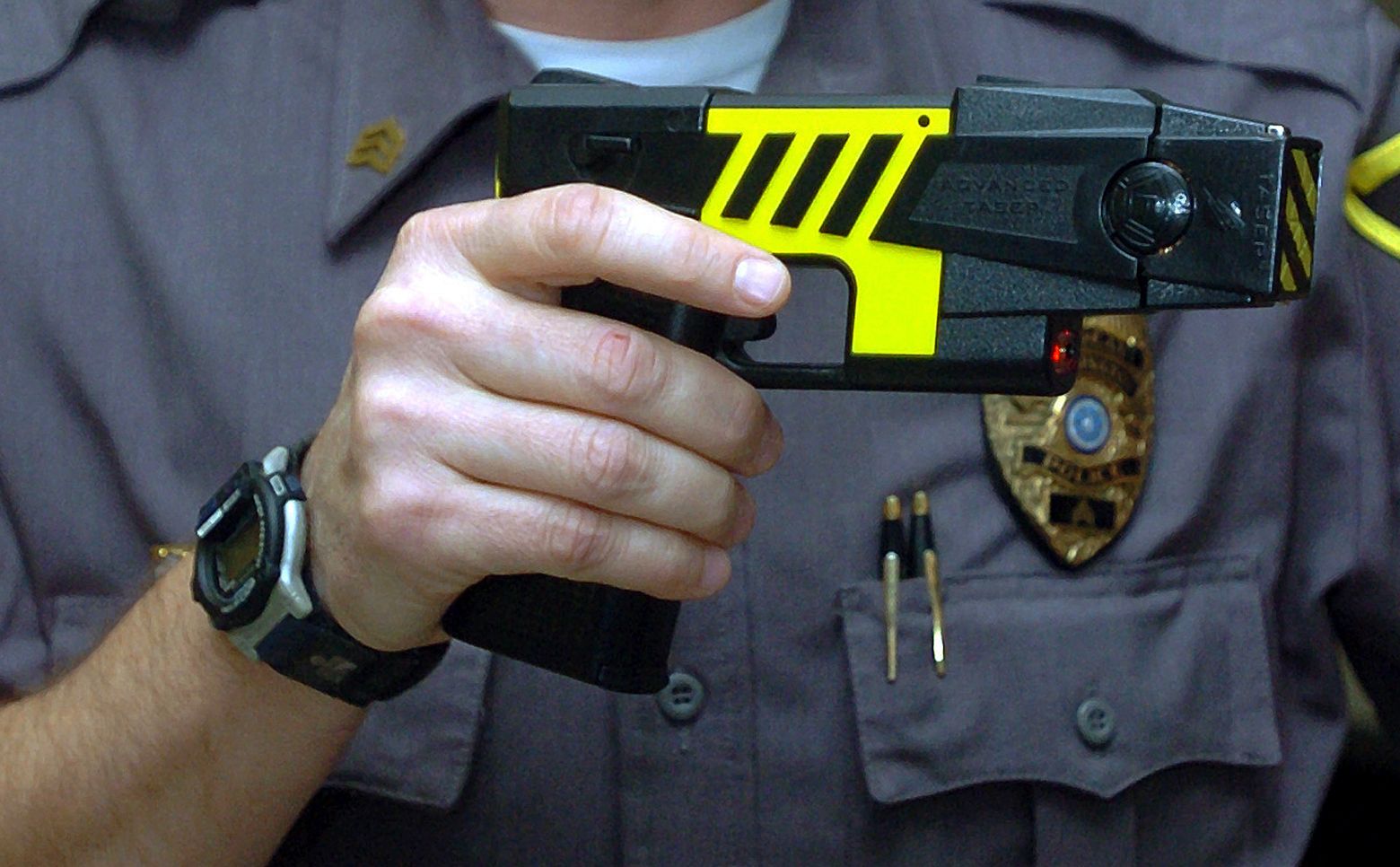The image is a close-up of a police officer's chest, focusing on his right hand holding a black Taser gun. The Taser, which is shaped like a pistol, features a distinctive bright yellow section in the middle with black lines and markings. Below the yellow section, a red light is visible, and the tip has a black square adorned with a diagonal yellow and black striped sticker. The officer is wearing a grey uniform with a gold badge and two pens in the pocket on the left side. Underneath his uniform, he wears a white undershirt. His watch, black with silver outlines, is seen on his right wrist. The officer's skin is light, and his nails are well-clipped. The high-quality image also captures the slightly darker grey buttons of the uniform and the white circle on the badge.